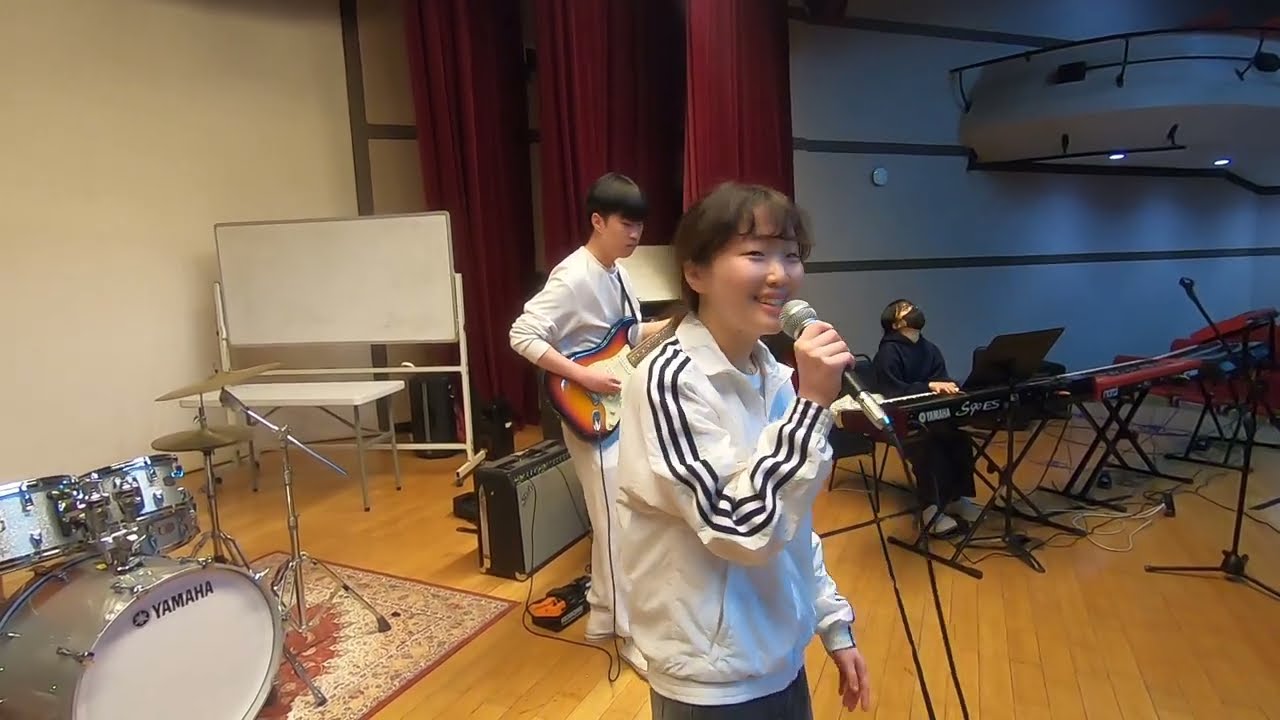The horizontally aligned rectangular image captures a scene inside a theater stage or similar indoor venue. The setting features white walls with three thin, horizontal stripes positioned at various heights on the right side, possibly in black or brown. In the foreground stands a young Asian woman, likely a teenager or in her early 20s, who is singing into a microphone. She has short brown hair pulled back with bangs and is wearing a white long-sleeve shirt adorned with three black Adidas stripes on the arms. The microphone she uses has a black handle and a silver top.

Behind her, a young Asian man wearing all white long sleeves plays a brown and white guitar with a black outline. Positioned slightly to the right in the background is another young Asian woman seated at a Yamaha keyboard, identifiable by the white writing on its black exterior. She is dressed in black attire with white shoes, wears a black mask, and is looking upward. Multiple keyboards surround her. 

To the left of the main action, a Yamaha drum set with two toms, a snare, a cymbal, a hi-hat, and a bass drum is visible but unoccupied. A portable chalkboard or whiteboard and an amplifier are also spotted near the drums. There is a red and tan patterned area rug on the floor, which resembles gym flooring, detailed with a brown brick-shaped pattern. Finally, a theater balcony is positioned at the far right of the image, suggesting the venue could be a stage for a music class, band practice, or performance in a high school or college.